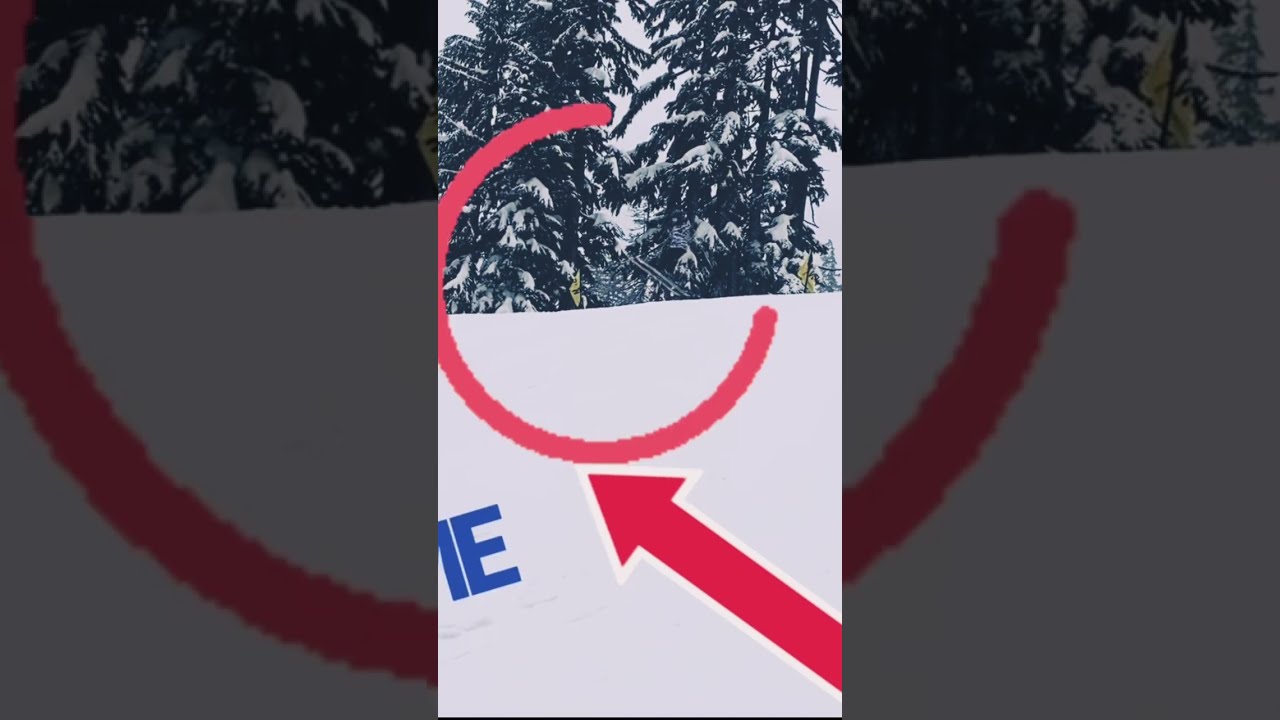The image appears to depict a snowy, outdoor winter landscape featuring evergreen trees with dark, black-green pine needles coated in white snow. Dominating the scene is a large red semicircle resembling the letter "C," located centrally and covering the base of the trees and an uneven layer of snow on the ground. A red arrow, outlined in white, points towards the open end of the semicircle. The sky is overcast, giving the impression of an impending snowfall. There are no people visible, enhancing the sense of a fresh, untouched snowfall. In the bottom left corner, the letters "IE" appear in blue, all capitalized. The image has the aesthetic of a simplified artistic rendition or a low-resolution, possibly digital, snapshot—reminiscent of a social media post, potentially from a platform like TikTok or Instagram.